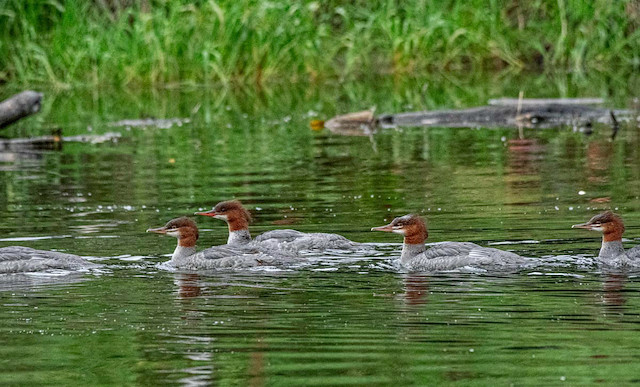This vibrant and lively image captures four ducks swimming in a horizontal row across a lake or pond, heading towards the left side of the frame. The ducks exhibit striking reddish-brown necks, with grayish-silver bodies and light brown beaks, complemented by a touch of black on the tops of their heads. The water, slightly wavy and greenish, hints at the ducks’ recent movements, adding dynamic energy to the scene. In the background, tall green grass or weeds rise from the water, and large sticks or pieces of wood float, contributing to a natural, almost swamp-like atmosphere. The photo is taken at a close range, suggesting the photographer was either in the water, on a dock, or utilized a zoom feature. The harmonious composition of the ducks and the serene, lush backdrop create a vivid snapshot of nature's tranquility.